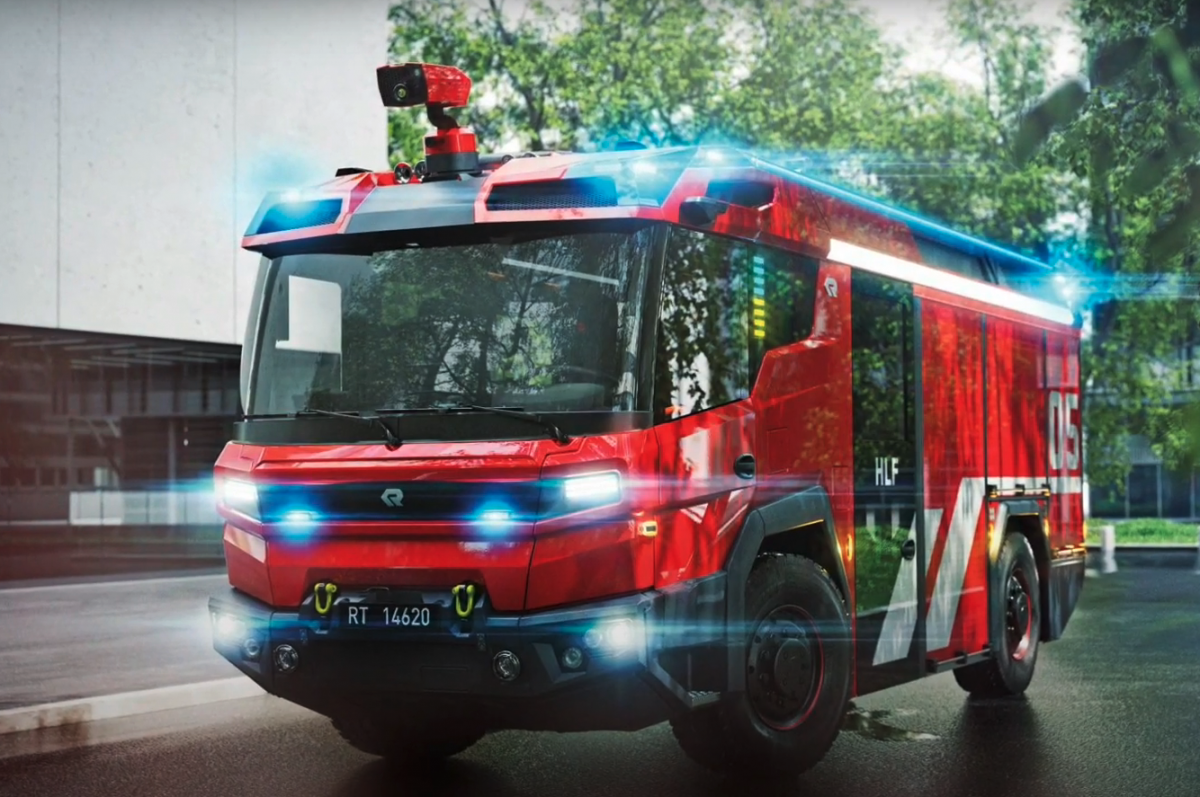This photograph captures a modern, bus-sized emergency vehicle, resembling a fire truck, primarily painted red with prominent white stripes and the number "05" marked on the side and rear. The vehicle features a large, slightly tinted wrap-around windshield reflecting nearby trees, obscuring any view of the interior. It is equipped with numerous blue and white flashing lights, contributing to a ghostly glow around the vehicle. A notable feature is a device on the roof that appears to be a camera or floodlight. The side door, labeled with "HLF," looks to be glass. The vehicle is parked on a blacktop surface next to a sleek, modern white office building with large windows, with more trees visible in the background. The license plate reads "RT-414629." The lights are on, though the vehicle seems stationary with no visible occupants or surrounding figures.